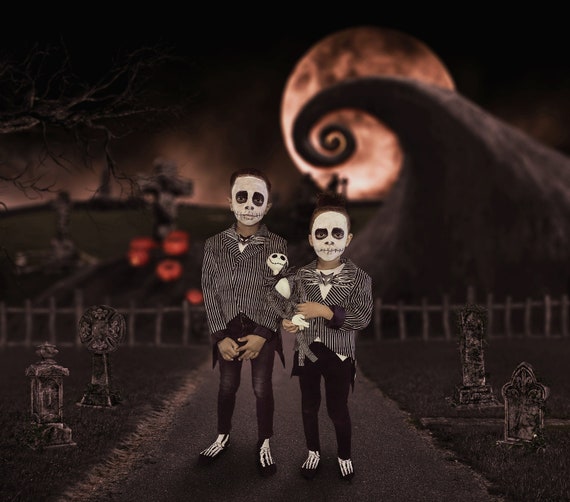Two children dressed in detailed Nightmare Before Christmas style costumes stand in the middle of a road, their appearance striking and skeletal. The taller child is on the left, and both wear black and white pinstripe suit jackets with black pants and skeleton-themed shoes or socks. Their faces are intricately painted: white base with black circles around their eyes and stitched lines over their mouths, evoking a skeletal look. Both wear skeleton masks, and the shorter boy on the right clutches a skeletal doll dressed similarly. 

They are surrounded by four grave markers, two on each side, and behind them lies a cemetery bordered by a gray fence. The background is dominated by a large moon partly obscured by the iconic swirling peak of a mountain, reminiscent of the Nightmare Before Christmas setting. There's also a tree trunk in the foreground, adding depth to the image. The overall scene is richly textured, blending elements of painting and drawing into a seamless collage-like style.